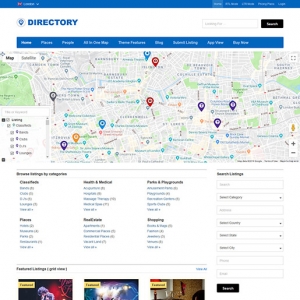At the top of the image, there is a blue header. Unfortunately, the text on the left and right sides is not legible. Below the blue header, there is a white section with the word "Directory" written in blue. To the right of this, there is a gray outlined search bar, and next to the search bar is a black button that says "Search" in white text. Below this, there is another blue bar with several menu items in white text, including "Home," "Places," "People," and "Site Map." Additional menu items are present, but they are unreadable.

Below the blue bars, there is a large gray map with various colored markers: purple, red, turquoise, gold, and black. The map is accompanied by a fine gray line, beneath which three categories are listed, showing locations and their respective counts. There are also three more categories at the bottom, each listing several items with numbers next to them. The map and lists are quite blurry and become more illegible when enlarged.

Another fine gray line follows with four black words that are not readable. Below this line, there are three partially cut-off images, each with a gold banner labeled "Featured." To the right of these images, there is a "View All" button in blue text.

On the right side of the image, there is an area to input text. The title above this area is in black text but is not readable. Below this area, there are eight labeled search bars, designed for inputting information. At the bottom, there is a black banner-like box with the word "Search" on it.